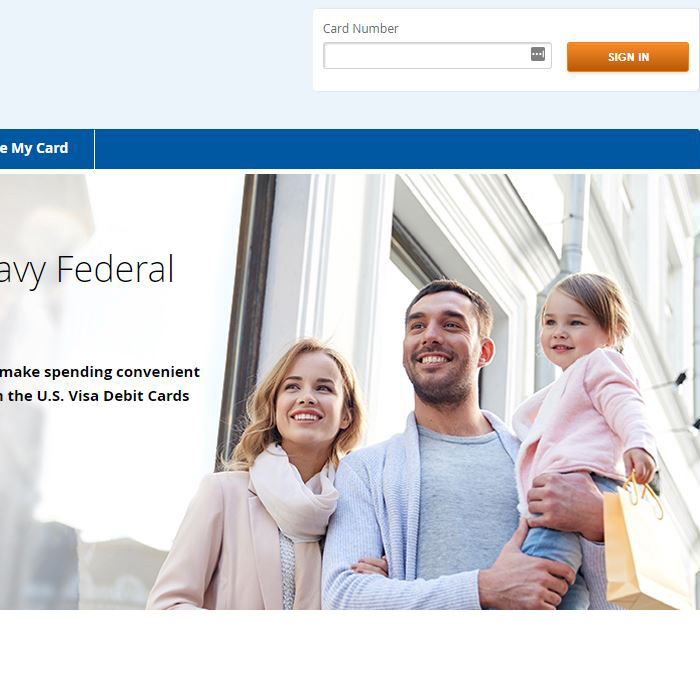The image captures a partially visible sign-in panel on what appears to be a user interface. The header of the panel is cut off, both on the upper right-hand corner and potentially on the left side as well. Prominently visible is a field for entering a card number, and below it is another input field. On the right side inset, there's a small gray square featuring three vertical dots and a vertical line. To the immediate right of this square is an orange rectangular button with white text that reads "Sign In."

Beneath the sign-in section, there is a small gap followed by a blue header bar. This header bar displays the partial text "my card," with only the letter "E" visible from the subsequent text, leaving the full header ambiguous.

The bottom portion of the image includes a stock photograph that has also been partially cut off. The photo depicts a family standing in front of a white building with large plate glass windows, likely in a shopping district. The family consists of a woman with either red or blonde hair wearing a pink sweater, and a man with short hair and a scruffy beard, dressed in a light gray cardigan. The man is holding a young daughter, who appears to be around two or three years old. She is dressed in a pink jacket and jeans, holding a small shopping bag.

Next to the family photo, some text is visible but partially cut off on the left. The legible text includes phrases like "make spending convenient," "U.S. Visa debit cards," and a possibility of "Navy Federal." The family in the image is smiling, creating a friendly and welcoming scene.